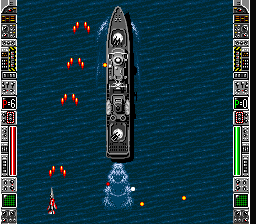The image resembles a dynamic scene from a video game, depicting a large gray battleship navigating through an ocean-like environment. The blue wavy background convincingly mimics the appearance of the sea. At the front of the battleship, a spray of water indicates its forward movement, with a larger spray trailing behind to emphasize its swift passage. Small, mysterious red objects, arranged in pairs, float intermittently in the water, their purpose unclear. On the opposite side, a few yellow dots can be observed, also scattered in the water. Flanking the screen on both sides are various vertical controls and interactive elements, suggesting the intricate gameplay mechanics of the scene.